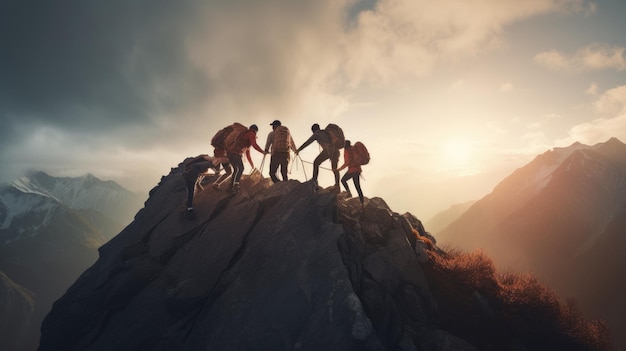The image captures six climbers atop a rugged, stone peak, the true focal point of the photograph taken from a distance. Each climber is equipped with hiking packs and joined by a guiding rope. The central figure, donning a black baseball cap, along with the others, directs their attention away from the camera. Their attire consists of jeans, jackets, hoodies, and warm-weather gear. The summit, characterized by rocky terrain and a touch of grass on its right slope, showcases the climbers seemingly having just reached the peak. In the backdrop, more mountain ranges extend with hints of snow peppering the rocky surfaces, creating a layered landscape. Above, the sky is filled with dense, white clouds mingling with hues of smoky blue, likely during sunrise, as sunlight partially pierces through the cloud cover to the mountains. Dark clouds loom to the left, suggesting an impending storm.